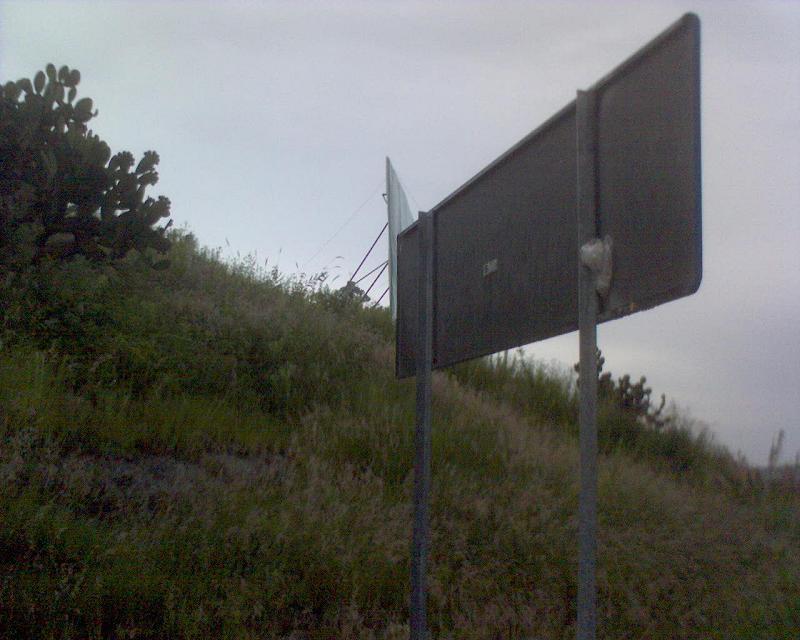This outdoor photograph showcases a gray sky filled with an assortment of white and gray clouds. Dominating the scene is a diagonal grassy hill, ascending from the lower right to the upper left, interspersed with varying shades of green and brown. At the top left of the hill, there are verdant cacti and a lush green bush. Below and toward the left, there are patches of gray and brown stones or dirt. Prominently featured in the middle of the photograph is the back of a street sign, supported by lighter silver metal poles and characterized by visible clips. Additionally, a large white billboard with zigzagging poles grounding it is positioned at the hill's summit, adding structure to the natural landscape.